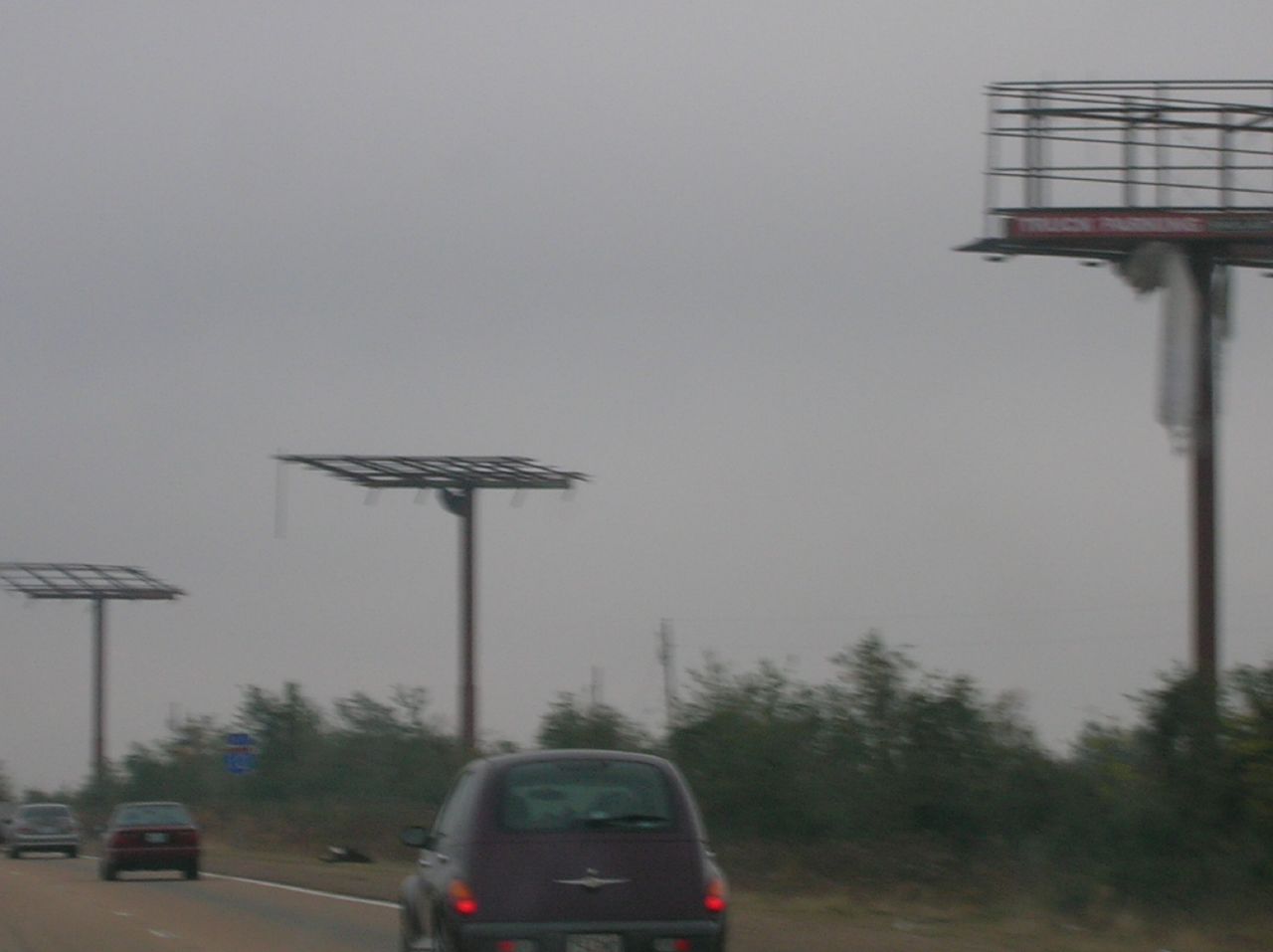The image depicts a roadway with distinct traffic markings, including a broken white line down the middle and a solid white line at the curb. The scene includes the rear view of three vehicles. The first, a dark brown PT Cruiser, has its taillights illuminated in red and features a visible back windshield wiper. A smaller, indistinct red car is in front of it, followed by one or two other vehicles that are barely visible.

In the background, there are several large, empty billboard structures. On the far right, one billboard stands upright with a faint, unreadable message that includes the word "truck." Another billboard in the center of the image lies flat, seemingly toppled by the wind. A third billboard structure in the distance is also collapsed. The backdrop includes a stretch of grass and scattered trees, framing the otherwise desolate roadway scene.